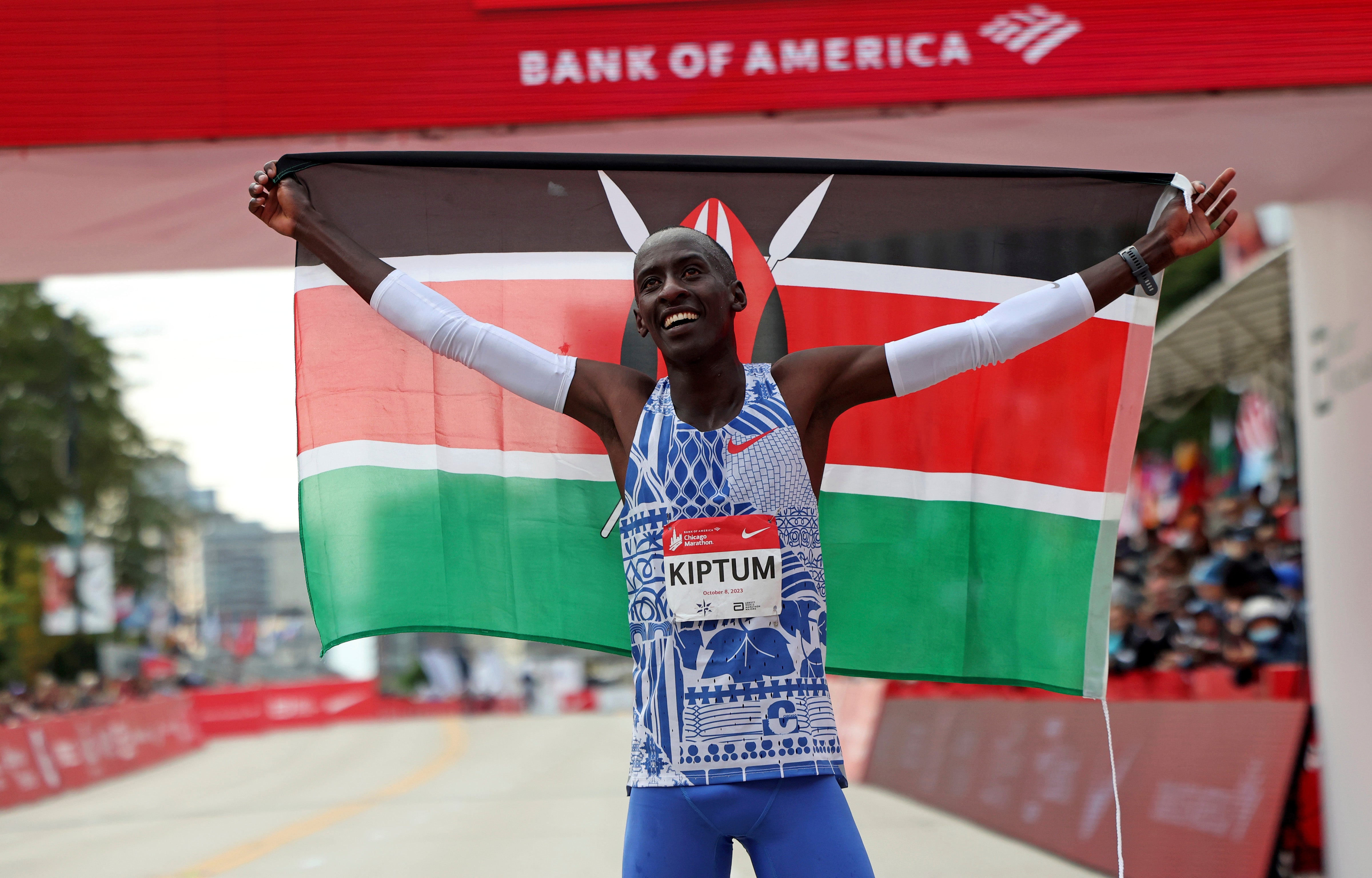In this photo, marathon runner Kiptum, sponsored by Nike, is seen celebrating his victory at the Bank of America Chicago Marathon. He stands triumphant with his arms raised, holding the Kenyan flag, which features horizontal stripes in black, red, and green, separated by thin white lines. Kiptum, who has dark skin and a shaved head, is dressed in a blue and white patterned Nike singlet, blue shorts, and white arm sleeves. He also wears a heart rate monitor on his left wrist. A red banner with the Bank of America logo hangs above him, marking the finish line. The background reveals a crowd of spectators, trees, an overcast sky, and buildings. Kiptum's jubilant smile and upward gaze capture the elation of his impressive achievement.